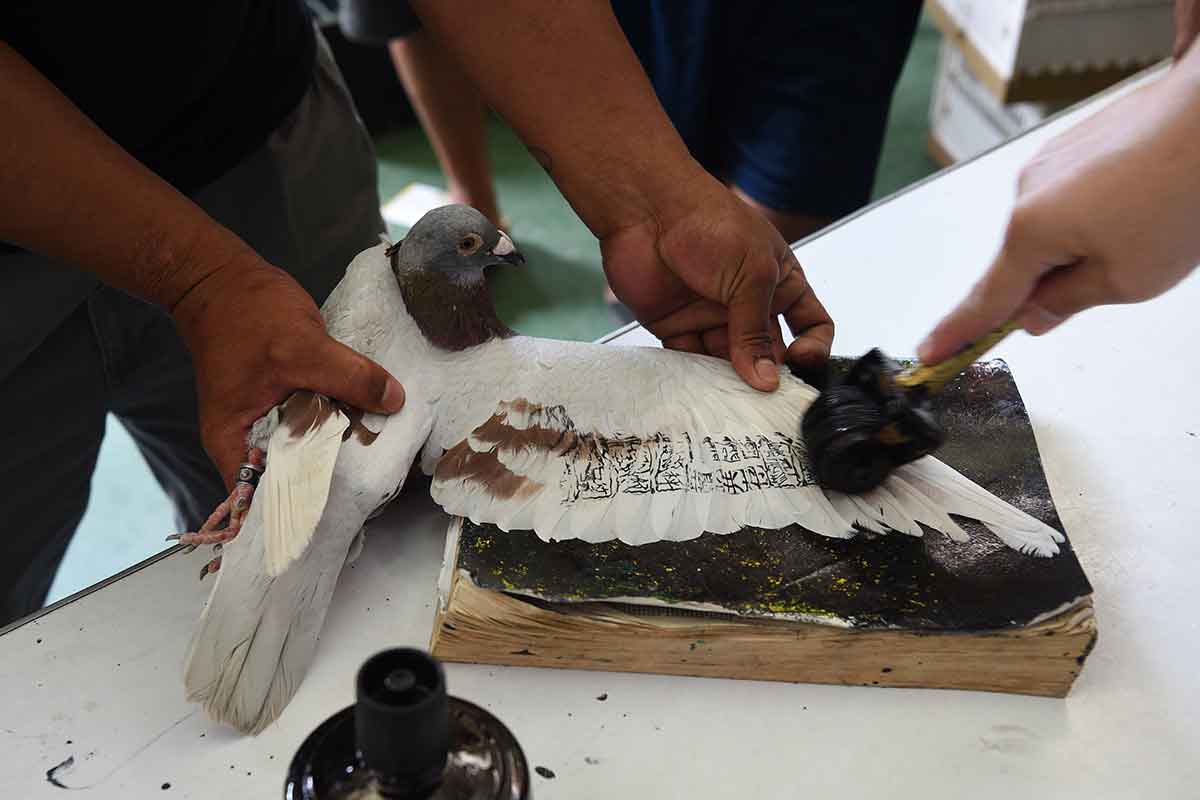In the image, two people's hands are visible as they work meticulously at a white workbench. The scene centers around a calm, white pigeon with a gray head, whose outstretched wing rests on an old, ink-stained book. The person on the left, whose dark brown hands are visible from the waist down, gently holds the pigeon in place, using one hand to keep the wing spread open. A lighter-skinned hand from the right of the frame carefully maneuvers a small ink roller across the pigeon’s wing, imprinting it with intricate, Japanese-like characters. Nearby, a black ink bottle sits on the table, with little splatters casting a subtle pattern on the smooth white surface. The focused coordination between the two individuals highlights the delicate nature of their work.